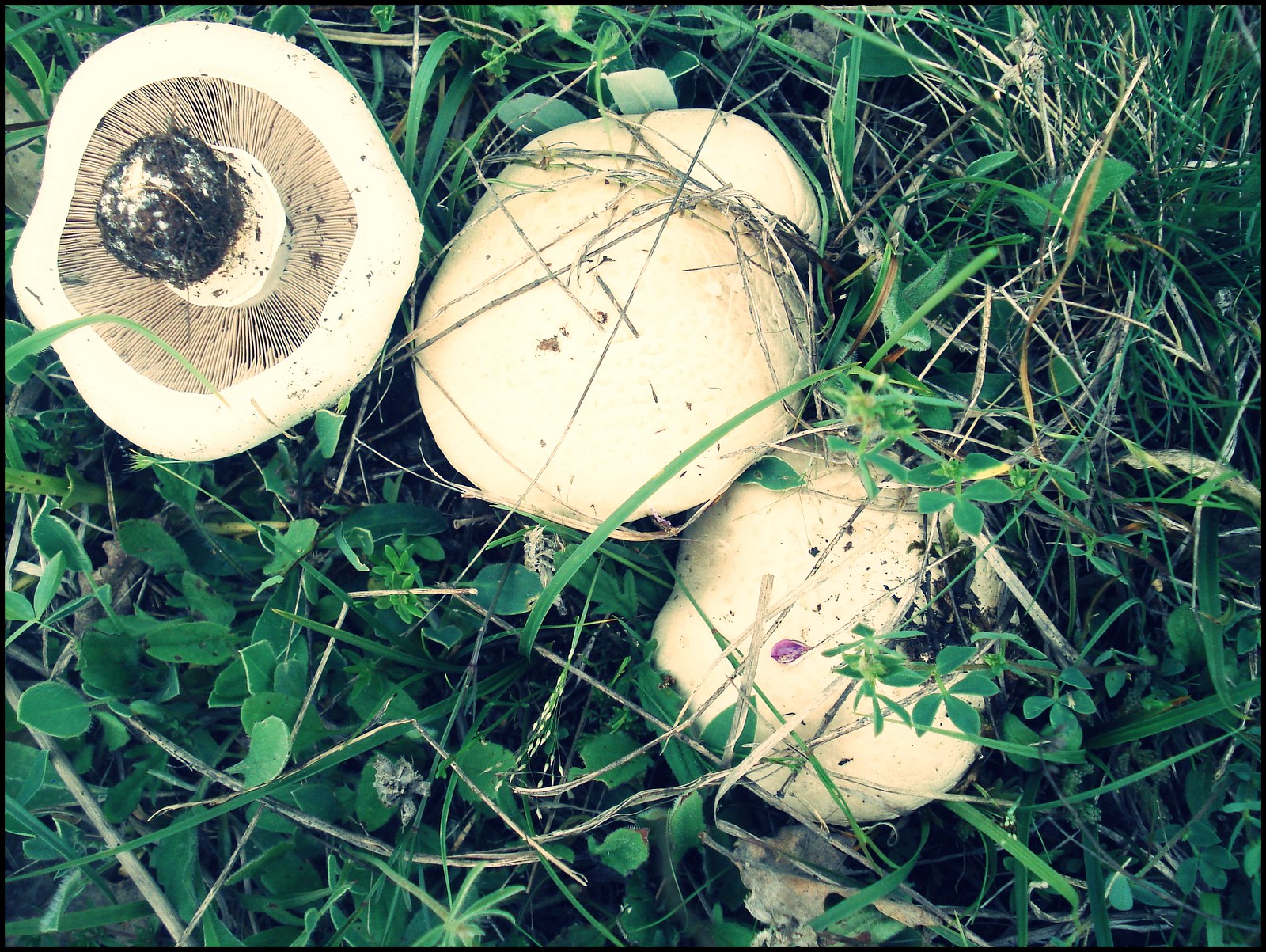In the image, a close-up shot reveals three mushrooms nestled among a dense, unkempt spread of long grass and clover, the scene seemingly from a field or possibly a backyard. The primary focus is on the mushroom caps, which are a delicate light brown to cream color, adorned with naturally occurring spots and specks of dirt. The two central mushrooms have long blades of grass draped over their caps, adding to their earthy charm.

Centered to the right, these two mushrooms appear closely grouped as though they have grown together in the ground. Their tops are dotted and slightly discolored, contributing to their wild appearance. To the top left of the photo lies a distinctive third mushroom, lying upside down. This upturned mushroom exposes its intricate, fine gills that line the brownish interior, and displays a dark gray, somewhat dirt-streaked stem, indicating it has been freshly pulled from the earth. Scattered across the grass are various small, round, and fat leaves, alongside some scattered flower petals, enhancing the rustic, natural vibe of the scene. 

Overall, the image showcases the raw, unmanicured beauty of these mushrooms surrounded by weedy, untrimmed grass and natural debris.